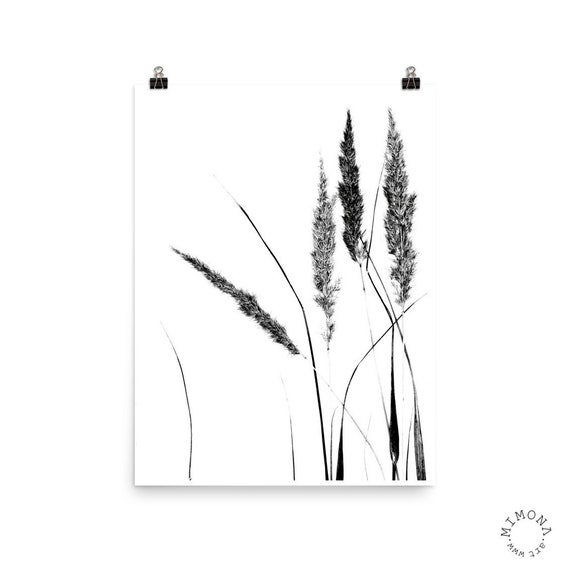The image portrays a minimalist black-and-white sketch of plant stems, resembling wheat or lavender, on a plain white paper fastened by two black binder clips at the top corners. The stems, concentrated more on the right side, feature intricate details of seed heads or grains that appear to weigh them down, with one bent and angled towards the left. Positioned on a white surface that creates a shadow behind, the sketch exudes a delicate balance between simplicity and detail. The bottom right corner of the surface bears the logo "Mimona MMM www.mimona.art," suggesting a possible digital manipulation or artistic presentation for an online gallery display.